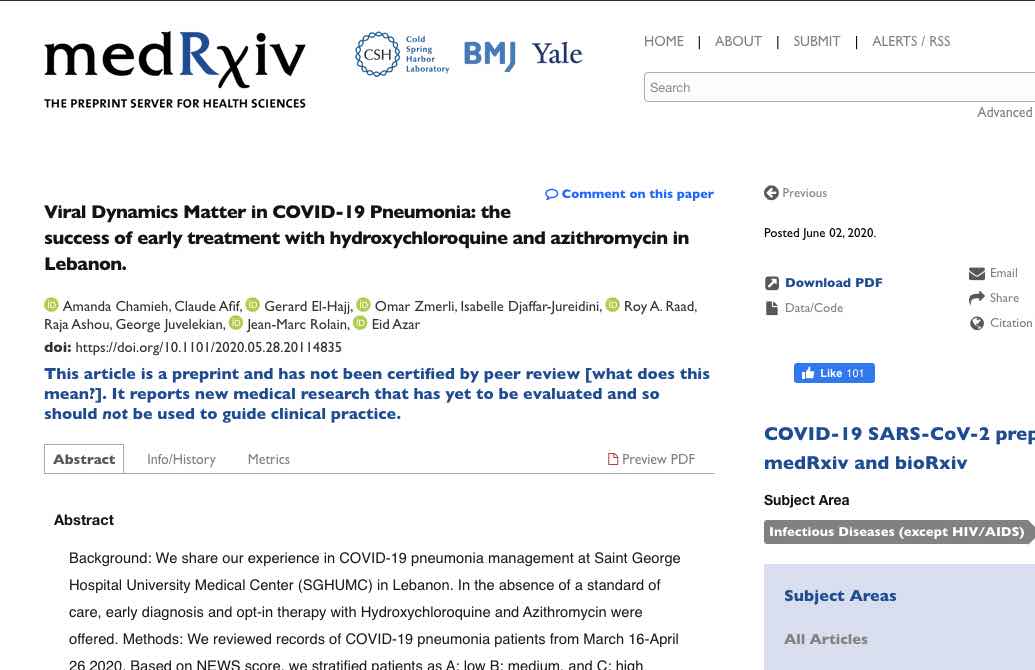Screenshot of a medRxiv webpage titled "Viral Dynamics Matter in COVID-19 Pneumonia: The Success of Early Treatment with Hydroxychloroquine and Azithromycin in Lebanon" posted on June 2nd, 2020. The screenshot shows the familiar interface of the preprint server for health sciences, displaying the logo of Cold Spring Harbor Laboratory encircled by chains, and partnerships with BMJ and Yale indicated in blue text. 

At the top of the page, navigation links are visible, including Home, About, Submit, and Alerts/RSS, along with a search bar and an 'Advanced' search button. The research paper is credited to several authors, each accompanied by a small green icon. 

On the right-hand side, user interaction buttons are displayed: 'Download PDF', email, share, citation, and data code buttons, along with a like button showing 101 likes. The page is categorized under COVID-19 and SARS-COV-2 research.